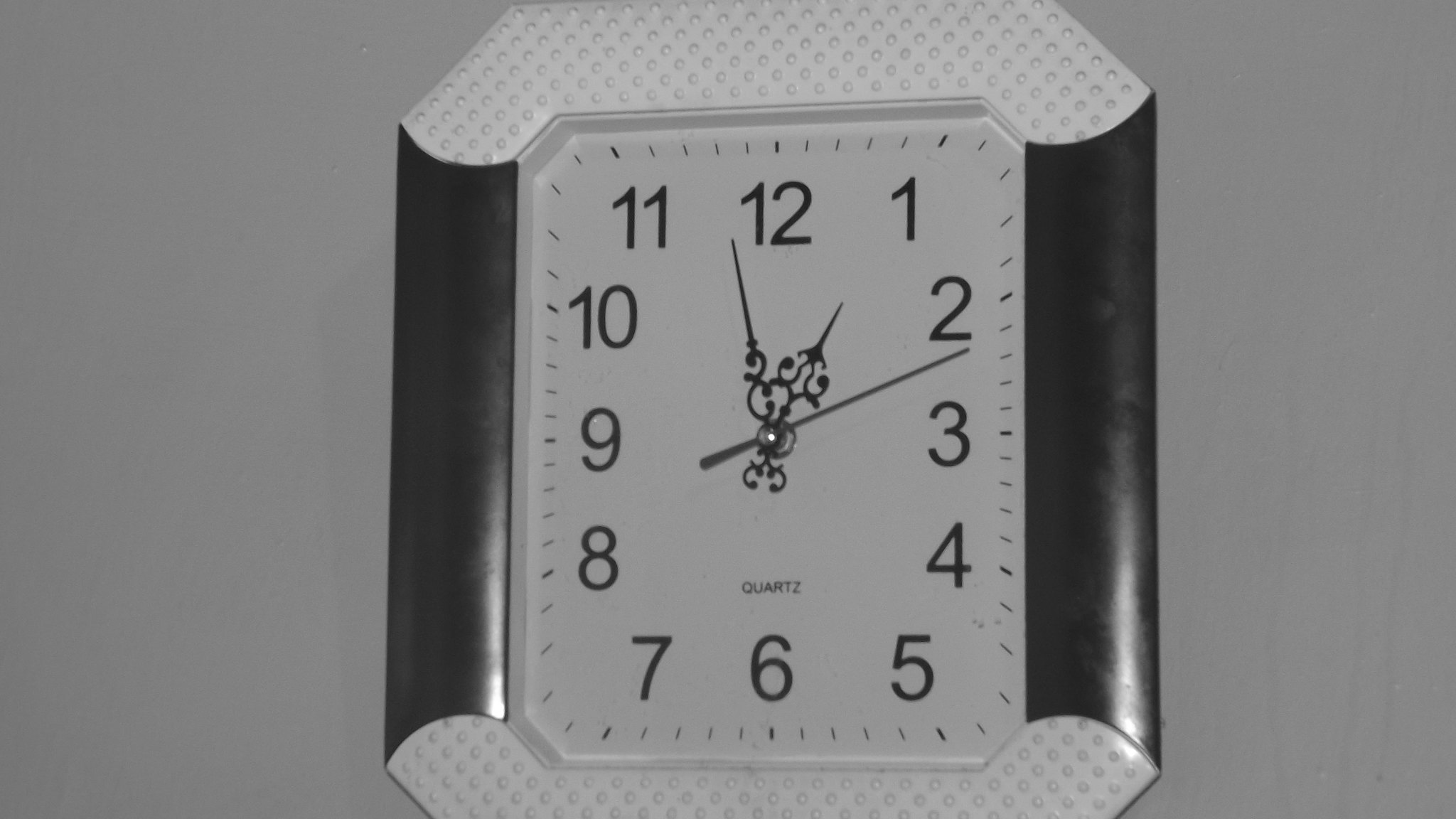A meticulously crafted image depicts a uniquely designed clock against a plain gray backdrop, giving it a somewhat surreal, computer-generated appearance. The clock is diminutive in size and roughly square in shape. Its top and bottom edges are adorned in a stark white color with a textured, bumpy surface reminiscent of Lego bricks, while the sides are sleek and black. Traditional Arabic numerals mark the hours, eschewing Roman numerals, and the word "Quartz" is inscribed on its face, indicating the type of movement. Adding a touch of intricacy, a delicate, flowery black design embellishes the clock's dial. As the hands point towards approximately 11:12, the hour hand stands out in black, while the minute hand gleams in silver, offering a striking contrast.